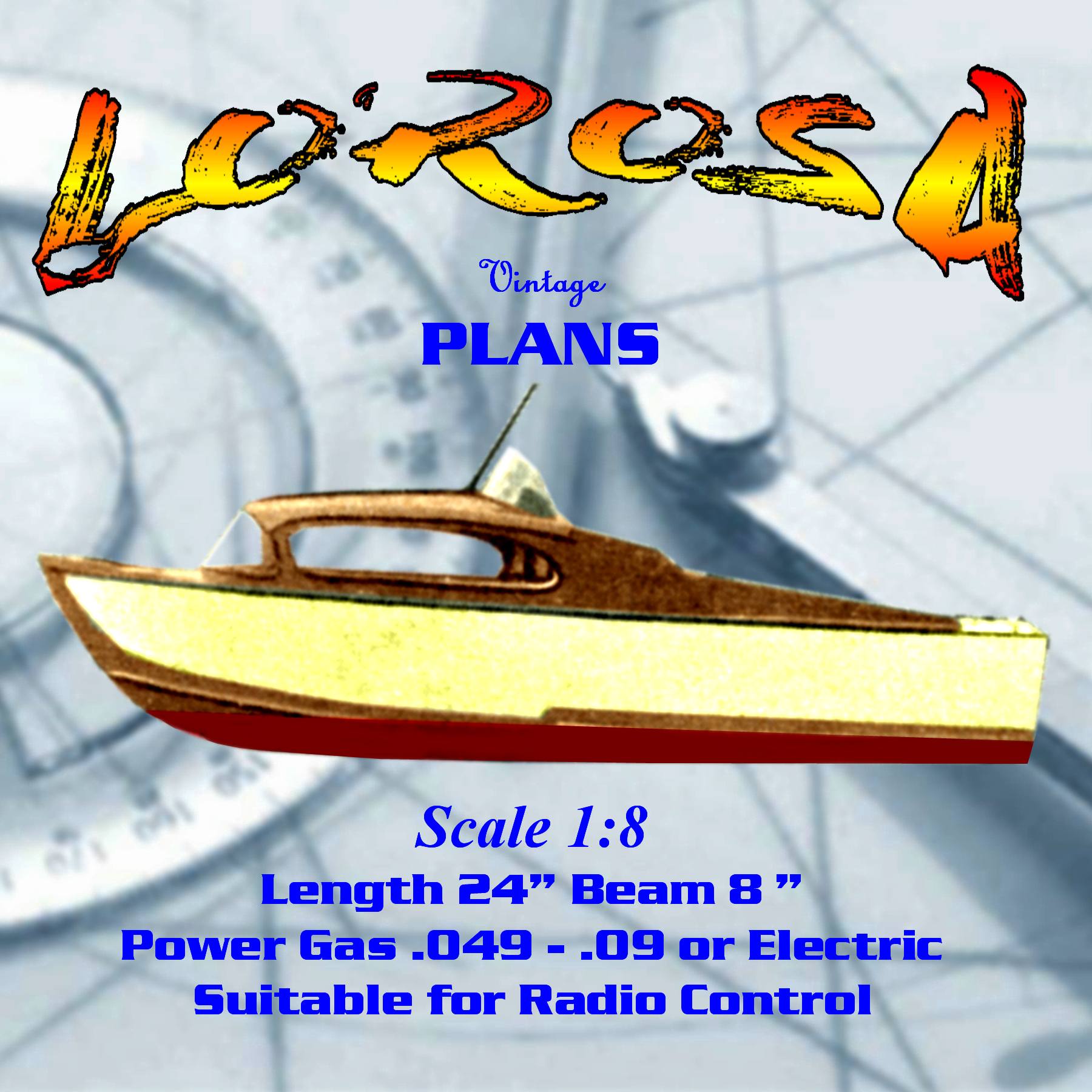The image is a detailed digital poster advertising a boat business. At the top, in a stylized red, orange, and yellow font, it reads "L-O-R-O-S-A" or "La Rosa." Below, in bright blue text, it says "Vintage Plans" in a combination of lowercase and all caps. The centerpiece is an old-style wooden motorboat facing left. It has a central white body, a wooden top, a dark antenna protruding from the roof, and a red keel. The cockpit has a light yellow window, and the boat's side is colored yellow with a maroon bottom. Overlaid text near the boat includes specifications: "Scale 1 to 8, Length 24 inches, Beam 8 inches, Power Gas .049 - .09 or Electric," indicating it is suitable for radio control. In the background, a circular shape, possibly a protractor design, symbolizes construction details. The text for these specifications is in a bright royal blue color.